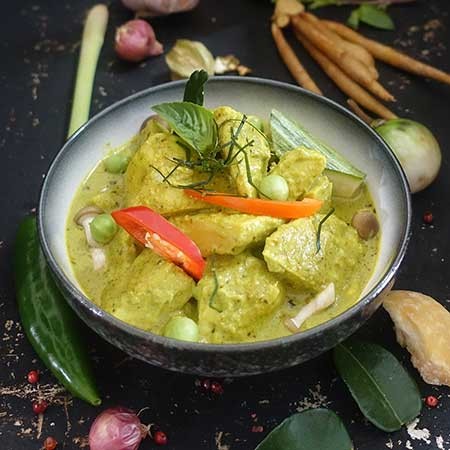The image depicts a vibrant bowl of food in a darker green stoneware bowl with a white interior, set on a black surface. The dish appears to be a vegetable curry or stew with a light greenish-yellow sauce. Visible ingredients include diced potatoes, peas, carrots, and slices of tomatoes, all garnished with sprigs of herbs and a single distinctive leaf. Surrounding the bowl on the table are various vegetables and ingredients, likely used in the dish: thin carrot-like vegetables in the back right, a long leek-like vegetable in the upper left, a shiny dark green vegetable in the lower left, and an onion just left of the bottom center. A few leaves are scattered just right of the bottom center. The surface is sprinkled with grains, red berries, and white specks, adding a textured detail to the composition. The arrangement and variety of elements contribute to a rich, appetizing presentation, highlighting the natural, colorful ingredients used in this seemingly ethnic culinary creation.